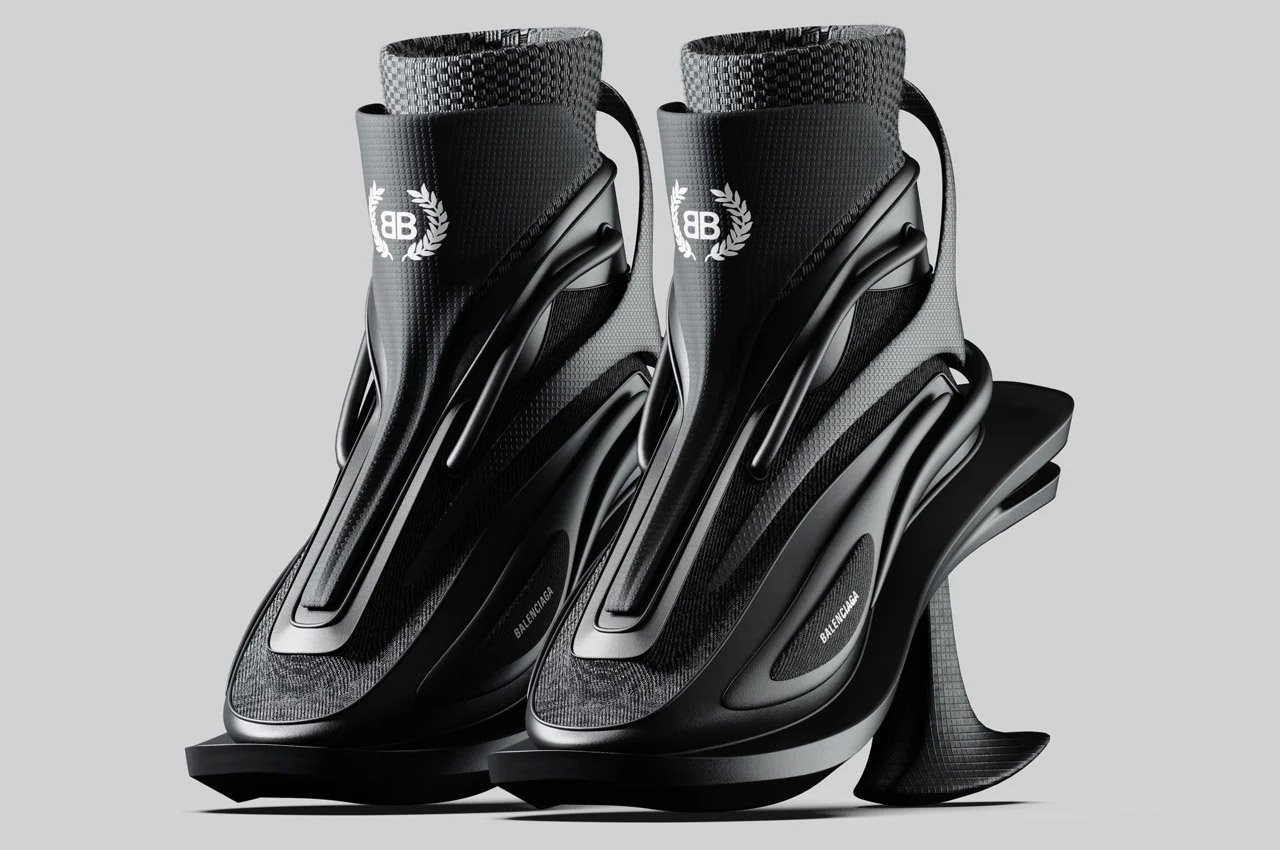In the photograph, there are two futuristic-looking black high heel shoes displayed on a raised stand. The shoes resemble a blend of high heel and sporty ski or snowboard boots, with a neoprene-like sleeve around the ankle and harder plastic around the top, ankle bone, and sole. These sleek, slip-on shoes feature a white logo on the front near the ankle area, consisting of two capital letter "B"s facing each other with curved, leafed branches around them, likely indicating a Balenciaga design. The unique high heels are set on a flat base with a prominent, thick spike extending from the back, making the shoes appear both avant-garde and functional. The stand is also black, accentuating the shoes' design and allowing a clear view of their innovative style.